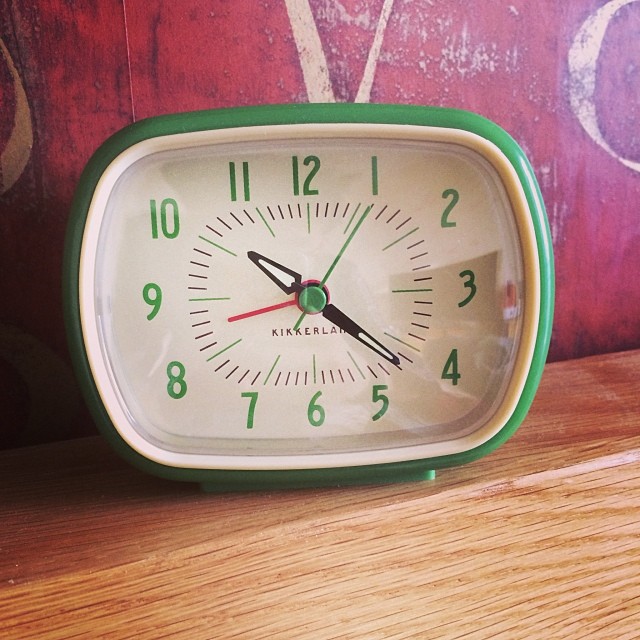This photograph captures a Kikkerland brand small tabletop analog clock with a distinct old-fashioned design. The clock, made of green plastic and shaped in a squat square form with rounded edges, features a white face adorned with green numerals. Its clear glass or plastic cover reveals black hour and minute hands, a green second hand, and a thin red alarm hand. The clock sits on a light-colored oak wood surface with a heavy grain, contrasting against a weathered, faded red wall in the background, which displays indistinct, off-white painted letters and markings. The overall scene evokes a nostalgic, rustic charm.